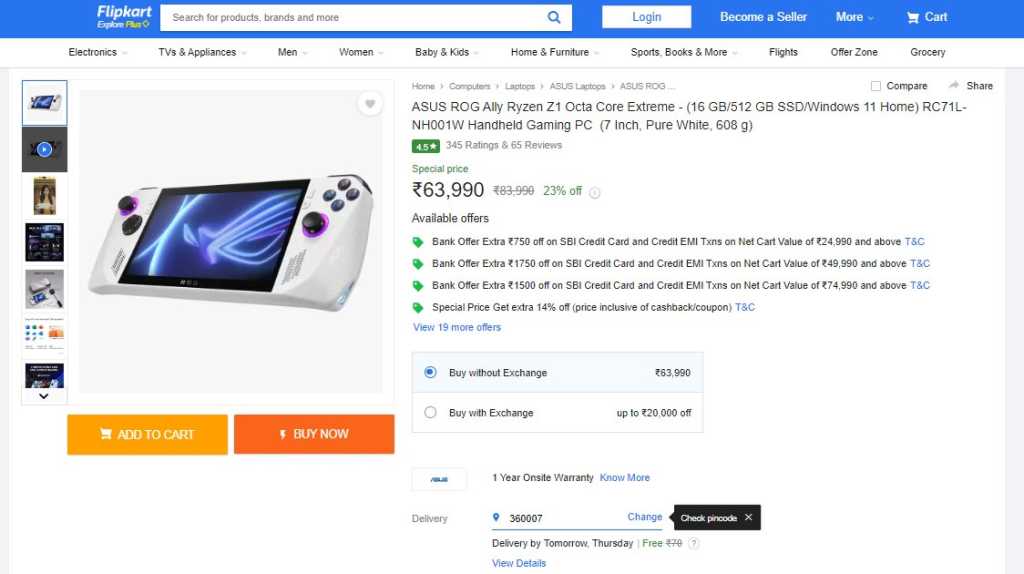The image depicts a Flipkart webpage, which prominently features the Flipkart logo at the top. Below the logo, there is a search bar flanked by options such as "Login," "Become a Seller," "More," and a cart icon. Further down, a comprehensive menu bar lists categories including Electronics, TV & Appliances, Men, Women, Baby & Kids, Home & Furniture, Sports, Books & More, Flights, Offer Zone, and Grocery.

In the main section of the page, a handheld gaming PC is highlighted. The featured product is the Asus ROG Ally Ryzen Z1 Octa-Core Extreme, positioned on the left side. There is a primary image of the handheld gaming PC accompanied by a vertical strip of smaller images showcasing different views, similar to the layout commonly seen on Amazon product pages.

To the right of the images, detailed information about the product is displayed. The device is priced at 63,990 yen, with a noted discount of 23% off. Below the price, there are prominent "Add to Cart" and "Buy Now" buttons in tangerine and orange colors, respectively.